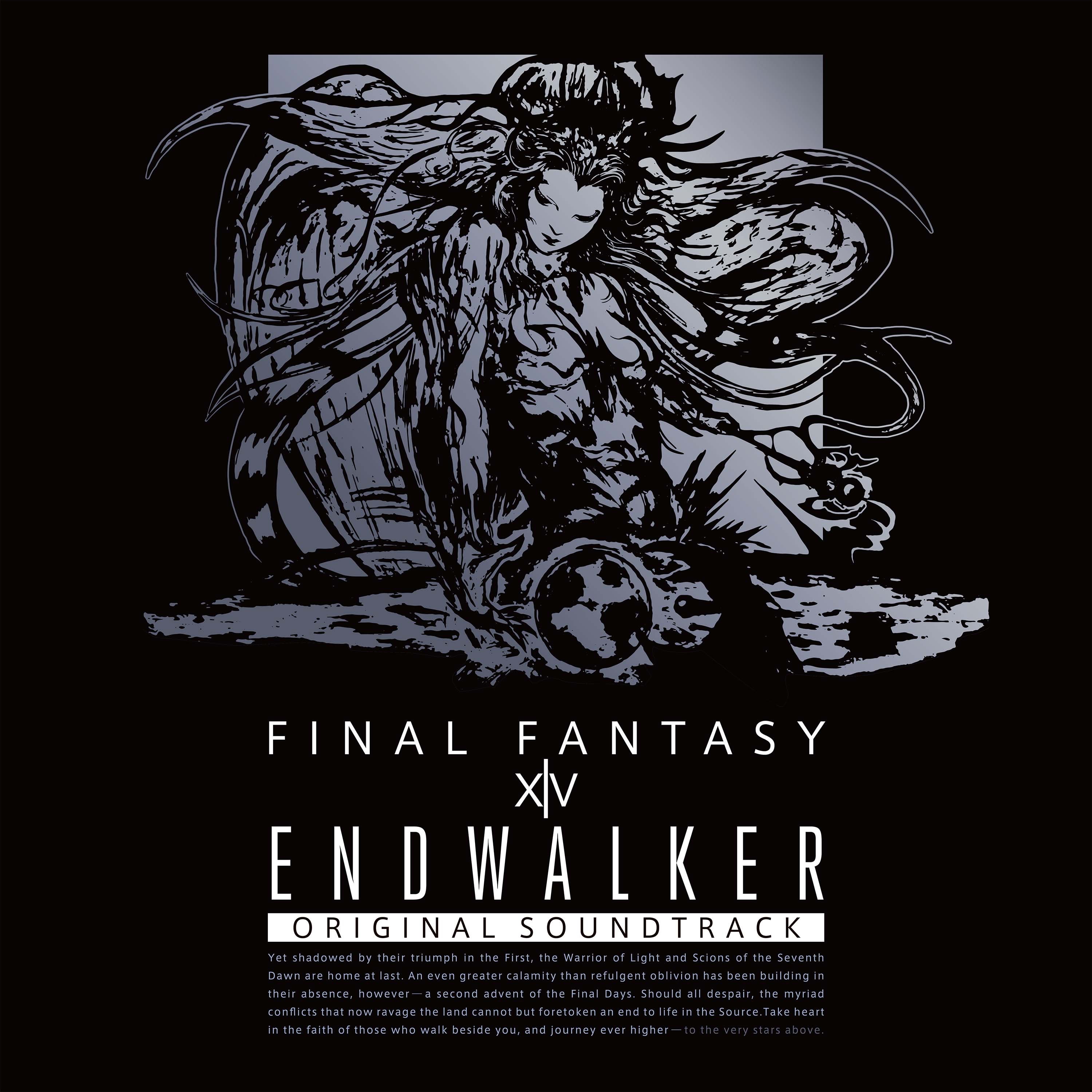This image is a square poster for the "Final Fantasy XV Endwalker Original Soundtrack." Dominated by a black background, the artwork features a striking illustration in silvery gray and black. The central figure is a stylized, shadowy female character with long, flowing hair that swirls in all directions, appearing to control the earth with a globe in her hands. Her elaborate form is both messy and splattery, adding a dynamic and powerful aesthetic to the piece. The title "FINAL FANTASY XV" is prominently displayed in white, all-caps font, with a vertical line between the X and V. Below it, "ENDWALKER ORIGINAL SOUNDTRACK" stands out, with "ENDWALKER" in white and "ORIGINAL SOUNDTRACK" in black lettering on a white horizontal rectangle. Additional text, written in a more faded white font, appears underneath the main title, contributing to the detailed and intricate design of the album cover.